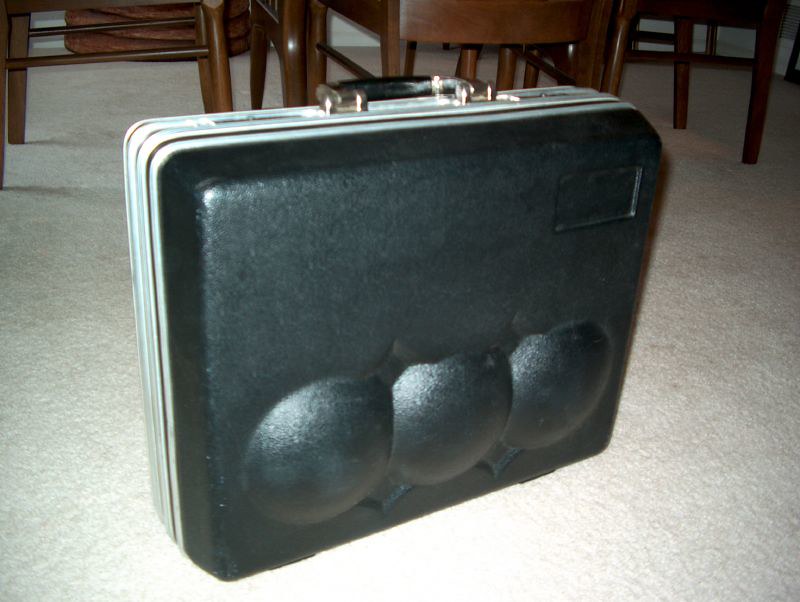In this peculiar image, a broadly rectangular, hard-shelled suitcase sits prominently on a cream-colored carpeted floor. The suitcase has a metallic, bluish-green-gray color that's worn in appearance, framed by a white or silver lining around its edges and a sturdy black handle. Notably, the side of the suitcase facing the viewer is matte black and features three raised, circular protuberances along the bottom, resembling rounded bubbles. There’s also a small, rectangular inset on this black side, to the right, whose purpose is unclear. In the background, dark wooden furniture, including a table and the legs of several chairs, suggests the setting is a conference or meeting room. The overall scene gives a sense of quiet, functional space, emphasizing the odd and distinctive details of the suitcase.